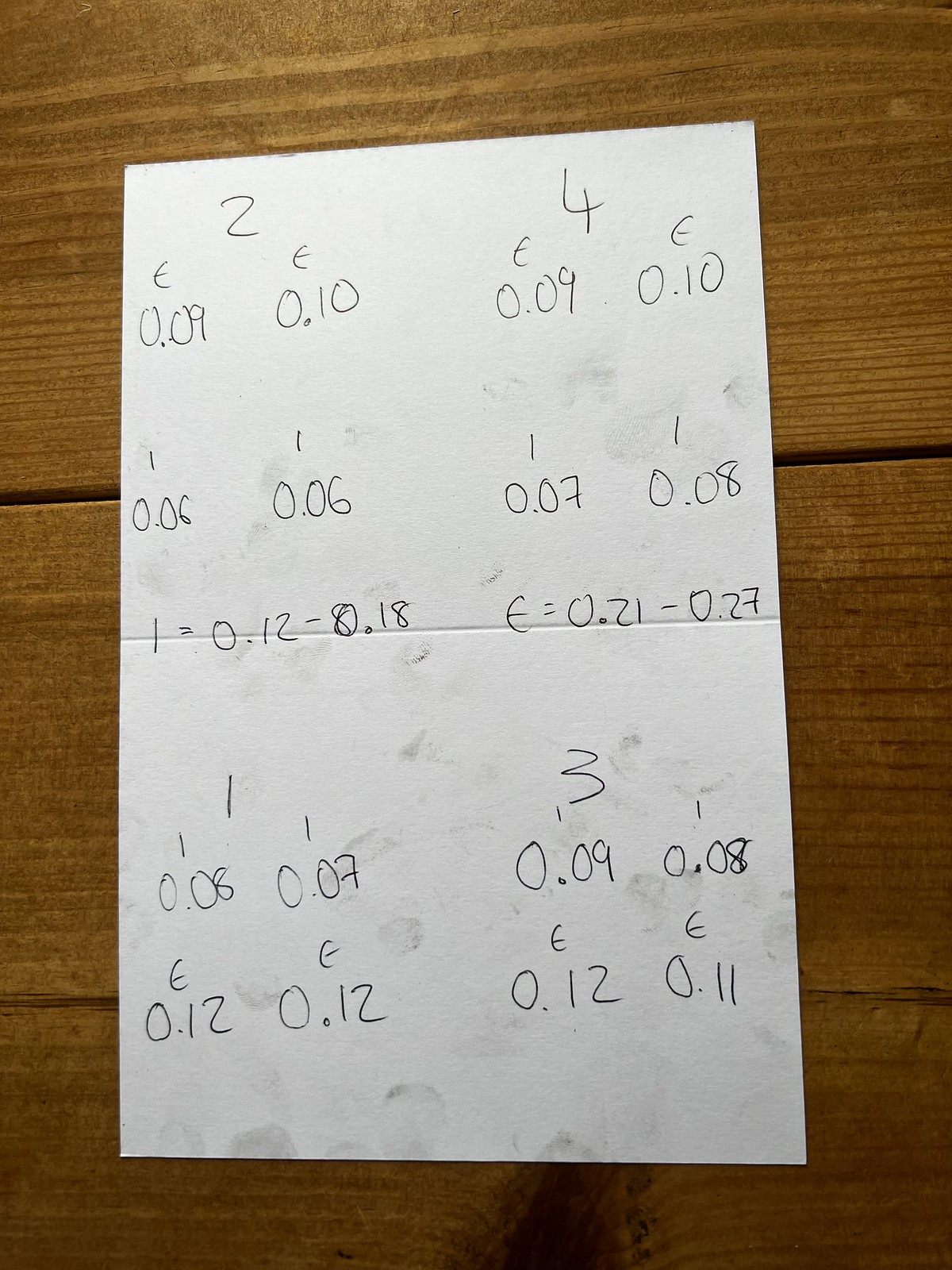The image presents a top-down view of an A4 piece of paper placed on a wooden table. The wooden table, made up of planks, features a distinct gap in the middle and a notable wood knot located at the bottom center. The wood grain runs horizontally from left to right.

The A4 paper is folded in half and positioned centrally on the table. A prominent crease line splits the paper, and it contains a detailed chart organized into two main sections, each comprising two columns and five rows.

In the top-left and top-right corners of the paper, the numbers "2" and "4" are written respectively. Below these numbers, the text includes symbols resembling either "e" or "£" signs and numerical values. Specifically:
- Top-left column: "0.09," "0.10"
- Top-right column: "0.09," "0.10"

Beneath these, the chart includes a row labeled with a "1" across:
- From left to right: "0.06," "0.06," "0.07," "0.08"

Further down, the paper displays equations:
- "1 = 0.12 - 0.18"
- "e = 0.21 - 0.27"

Another section appears with new columns, also spanning five rows. At the bottom left middle of this section is the number "1" and on the right side, the number "3."
- Below these numbers, under labels "1111": "0.08," "0.07," "0.09," "0.08"
- Further down: "ee, ee, 0.12, 0.12, 0.12, 0.11"

The paper's content appears to involve mathematical or statistical data, possibly calculations or a dataset represented in tabular form.